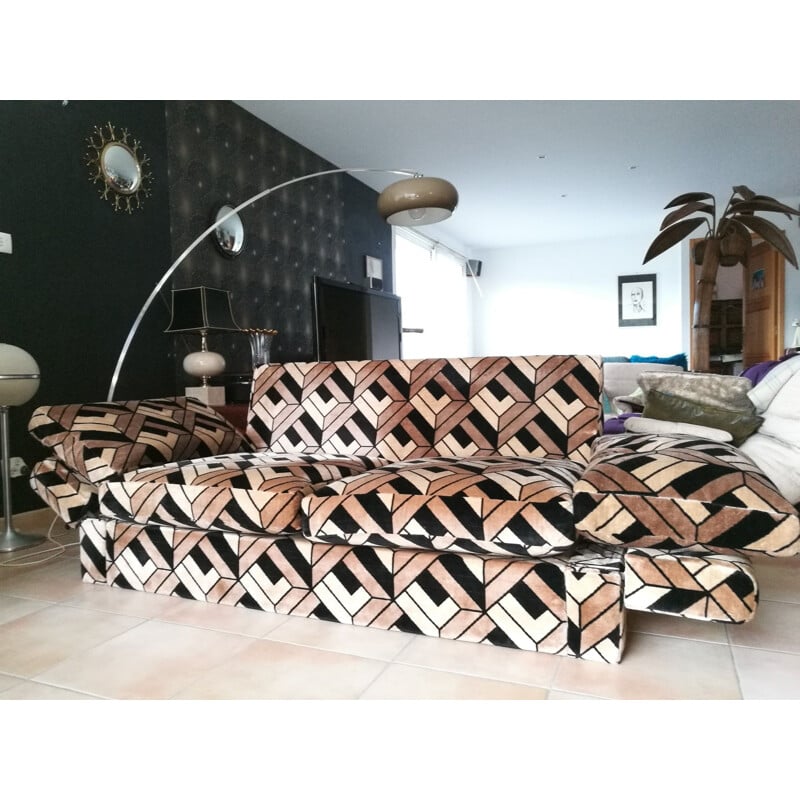In the photograph of a living room, the focal point is a detailed, patterned couch positioned centrally. The couch displays an intricate design with a combination of brown, beige, and black geometric shapes, resembling a stained-glass effect due to the black outlines around the shapes. It features both side cushions and an interesting skirt with a motif of larger brown squares merging into smaller beige squares. Adjacent to the left of the couch, a prominent arc-shaped lamp with a white and silver arm and a cylindrical beige shade is visible, revealing a bit of its white bulb. Next to this is another lamp distinguished by its square black shade, thin golden neck, semi-flattened white oval, tapering brass cylinder, and white square base. 

On the wall above the couch are two circular mirrors: one with a brass outline and decorative branches emanating from it, and the other with a simpler black metal frame. A partially visible large window in the background floods the room with sunlight, highlighting a fake palm tree with a round trunk and large green leaves nestled between the window and the couch. Across from the palm tree on the wall is a hand-drawn portrait of a man in a frame, and there is an open doorway with a large round door to the further right. The room's flooring is tiled, and the walls are white with one contrasting black wall featuring a distinct design. The photograph’s angle from a lower perspective accentuates the couch’s velour-like texture and the mid-century style of the hanging lamp.